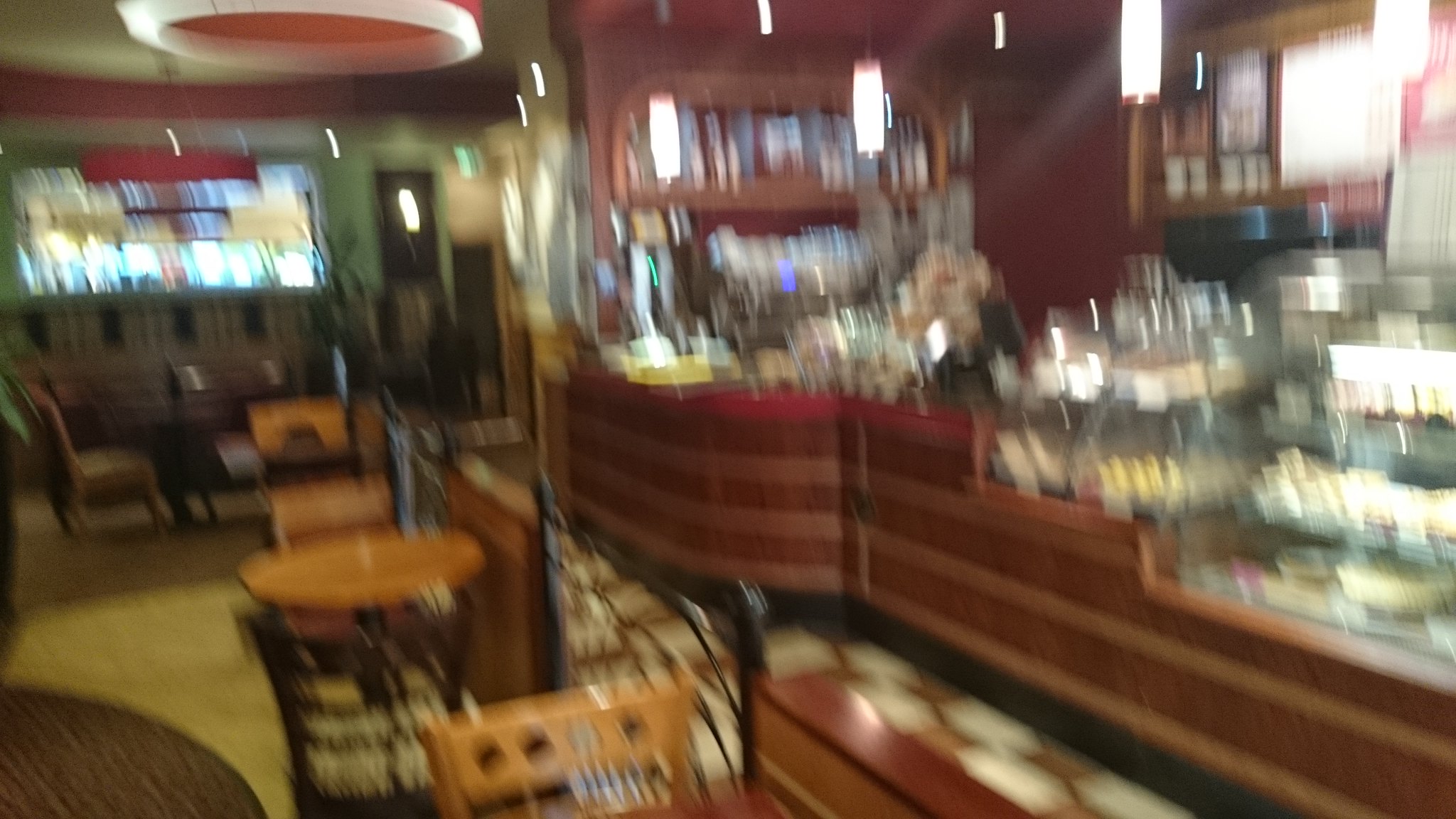This is a very blurry photograph of a casual coffee shop or bakery. On the left side of the image, there are several light brown, circular wooden coffee tables held by black pillars, each accompanied by matching wooden chairs with dark or blackish backs. The tables and chairs are spread out in what appears to be the dining area. On the right side, there is a coffee bar with a glass display case showcasing a variety of desserts and pastries, potentially including pies. The coffee bar is made of a long wooden structure and has overhead hanging lights with single light bulbs. Overall, the interior is predominantly brown with some white accents, and there is a door visible in the background. The coffee shop looks empty with no people present in the image.